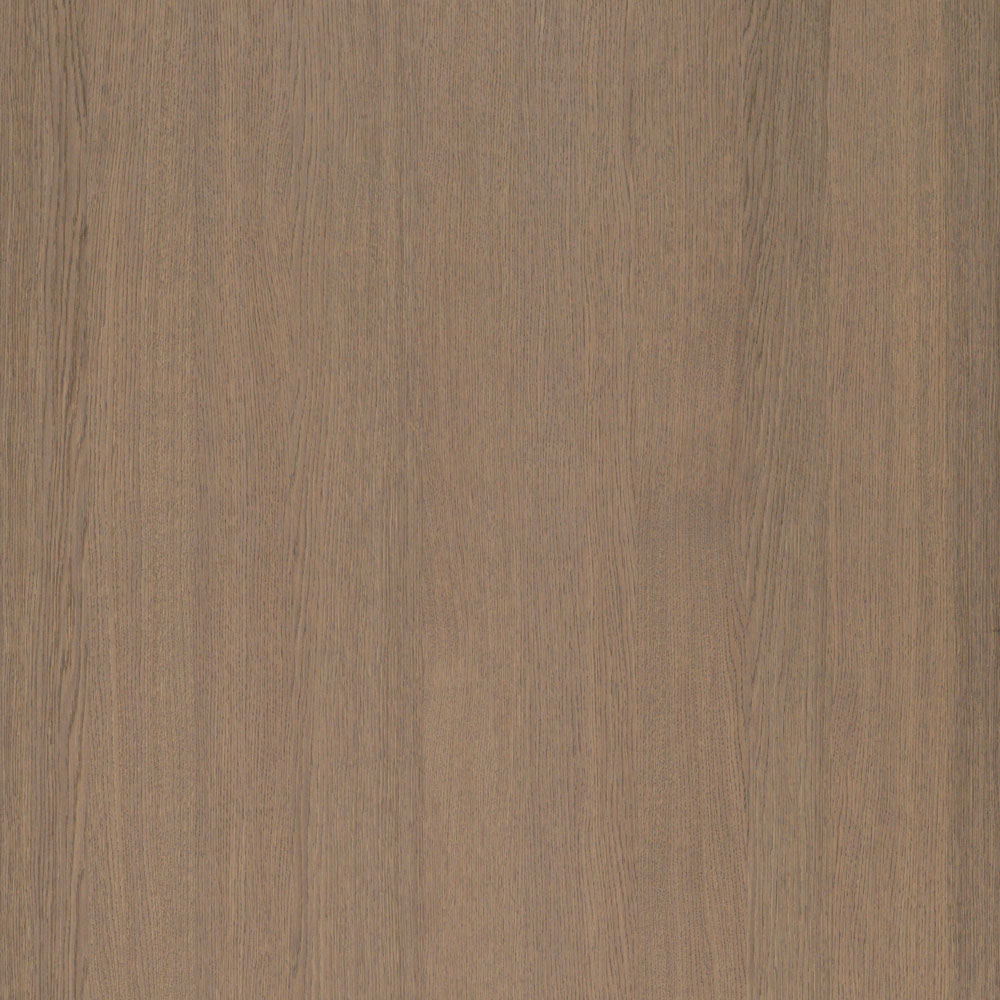This image features a detailed, close-up view of a wooden texture that takes up the entirety of the frame. The wood appears smooth and polished, suggesting it might be part of a piece of furniture or even a tabletop. The grain pattern is finely detailed with slight striations running vertically, displaying a variety of brown and black shades. The texture looks very uniform, with no visible knots, and the wood appears to be a lighter, perhaps oak color. The symmetrical composition and consistent texture indicate that this may either be a real wooden surface or a high-quality vinyl imitation, possibly showcased as a sample from a home improvement store. There is no text or other objects present, making the intricacies of the wood grain the primary focus.